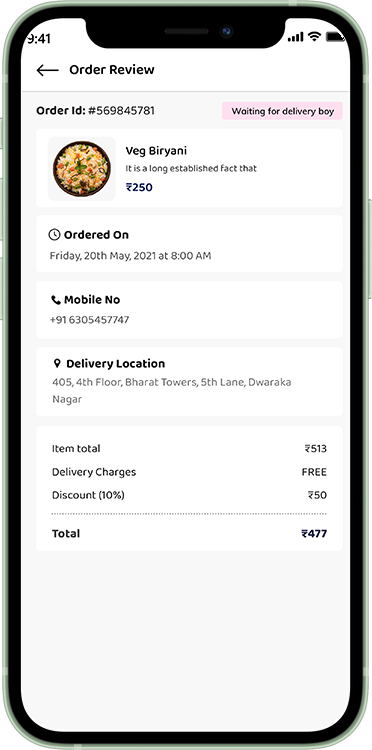The image showcases a smartphone with a mint green border case. The left side of the phone features three mint green buttons, while the right side has one button of the same color. Surrounding the screen is a black outline. At the top of the phone, there is a small circle, likely the front camera, and a barely visible oval, which might be the speaker.

The phone's display shows a white background with various details. In the upper left-hand corner, the time is displayed as 9:41 AM in black text. The status bar indicates three bars for Wi-Fi and four bars for cellular reception, suggesting excellent connectivity. The battery icon appears mostly full but is partially cut off.

Beneath the status bar, a navigation arrow pointing to the left is visible, next to the screen title "Order Review" written in capital letters and black text. Directly below, a gray line stretches across the screen, under which "Order ID #569-845-781" is printed in black.

Further down, within a large rectangular section, the text reads "Wait for delivery, boy," followed by "Vague Biryani." The currency details are unclear but are noted in blue as 250 units. Additional details include:

- Order date: Friday, 20th May 2021 at 8 AM.
- Mobile number: +91 63054 57747.
- Delivery location: 405, 4th Floor, Bharat Towers, 5th Lane, Dwarakanagar.
- Item total: 513.
- Delivery charge: Free.
- Discount applied: 50, resulting in a total of 477.

This thorough visual description provides a comprehensive overview of the phone and the displayed order details.